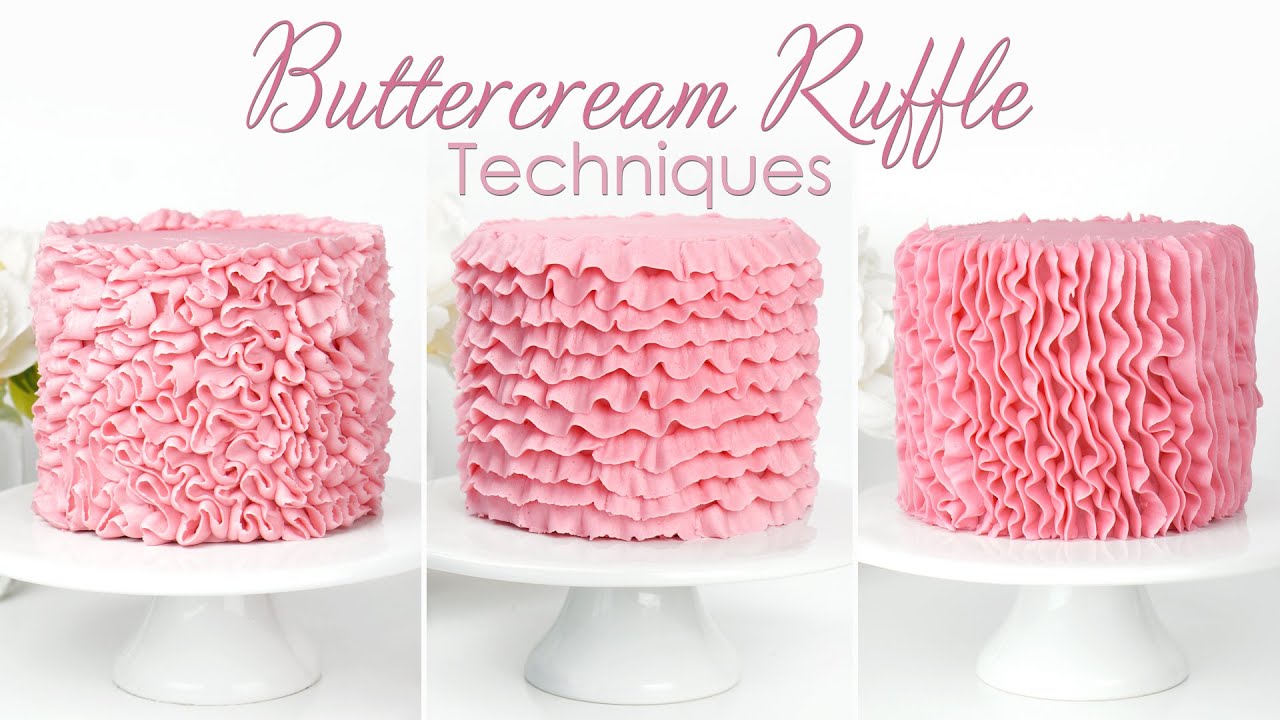The image showcases a poster titled "Buttercream Ruffle Techniques" written in pink script at the top, featuring three side-by-side photos of cakes adorned with pink buttercream ruffles. Each cake sits on a white pedestal cake stand against a white background with subtle greenery in the distance. 

The first cake, positioned on the far left, exhibits tightly grouped, wavy ruffles resembling brain sulci, providing a dense, intricate texture. The middle cake displays evenly spaced ruffled rings, akin to the end of a skirt, creating horizontal rows that encircle the cake. The rightmost cake showcases vertical lines of ruffles, producing a distinct up-and-down pattern. All three multi-layered cakes have smooth, flat tops, emphasizing the elaborate ruffle work cascading down their sides.